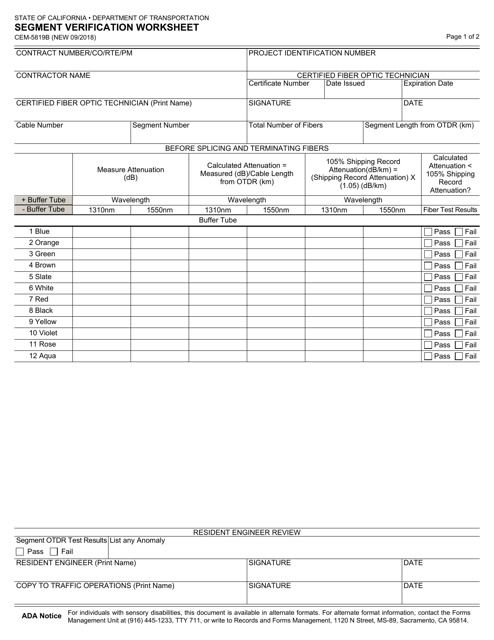The image showcases a worksheet from the State of California Department of Transportation. Titled "Segment Verification Worksheet," the document appears to be from the year 2018 with a reference identifier "new 09-2000." This is page 1 of a 2-page form, written entirely in black font. 

The upper section includes labeled fields for "Contract Number," "Project Identification Number," "Contractor Name," "Certified Fiber Optic Technician," "Certificate Number," "Date Issued," "Expiration Date," with all text boxes remaining blank. Below, there are fields for "Cable Number," "Segment Number," "Total Number of Fibers," and "Segment Length from OTDR" (Optical Time-Domain Reflectometer). 

A subsection titled "Before Splicing and Terminating Fibers" follows, featuring various sub-menus with measurements for alteration, both measured and calculated, though the content is difficult to read. The fields for "Buffer Tube" contain rows of blank boxes tailored for input, each associated with colors such as blue, orange, green, brown, slate, white, red, black, yellow, violet, rose, and aqua. Nearby are "Pass" and "Fail" checkboxes, none of which are marked.

The document further includes a section for the "Resident Engineer Review," with headings like "Segment OTDR Test Results - Pass or Fail," which is also unfilled. It prompts for listing any anomalies with spaces for the resident engineer's printed name, signature, and date, as well as copying the results to traffic operations.

At the bottom, an ADA notice informs individuals with sensory disabilities about the availability of the document in alternate formats, providing contact information for the Forms Management Unit, complete with a phone number and postal address: Records and Forms Management, 1120 North Street, Sacramento, California.